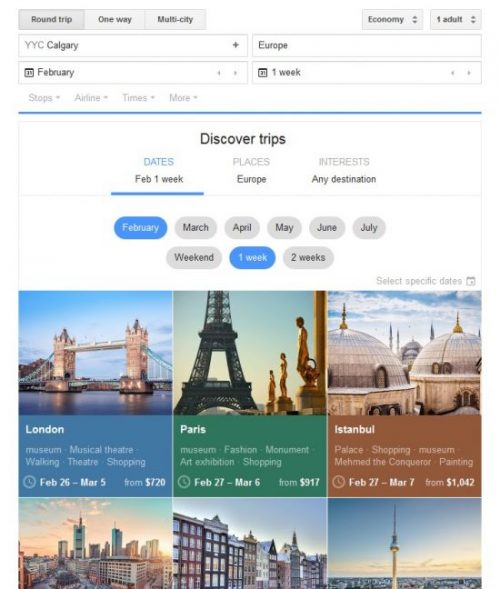The image showcases a detailed flight search interface with various options and settings. At the top left, there are three gray tabs labeled "Round Trip," "One-Way," "Multi-City," and an unlabelled black tab. Below these tabs, there are two outlined rectangles filled with white. The first rectangle reads "YYC Calgary," with the spelling "C-A-L-G-R-A-Y" indicated. Directly below, it displays "February."

On the top right of the first rectangle, there is a plus sign icon. Beside these, two gray side-by-side tabs are visible, with the first tab reading "Economy" in black and the adjacent one indicating "1 Adult." Below these tabs, two more outlined rectangles filled with white appear. The first rectangle shows "Europe" with a capital "E," and underneath, it specifies "1 Week."

Further down on the left, there are four words listed: "Stops," "Airlines," "Times," and "More." A thin blue line stretches across the interface, above a section where a white rectangle bordered in gray resides. In the center of this rectangle, "Discover Trips" is written in black.

Underneath "Discover Trips," on the left, there are date options highlighted in blue text with "Feb" (February) followed by "1 Week" in black with a blue underline. Adjacent to this in gray, the word "Places" in black is displayed, with "Europe" listed underneath. Further to the right, the gray word "Interest" is present, with "Any Destination" noted below.

At the bottom of the interface, there is a series of oval buttons. The first oval is blue, displaying "February" in white text, while the remaining ovals are gray, each labeled with the names of the following months: March, April, May, June, and July.